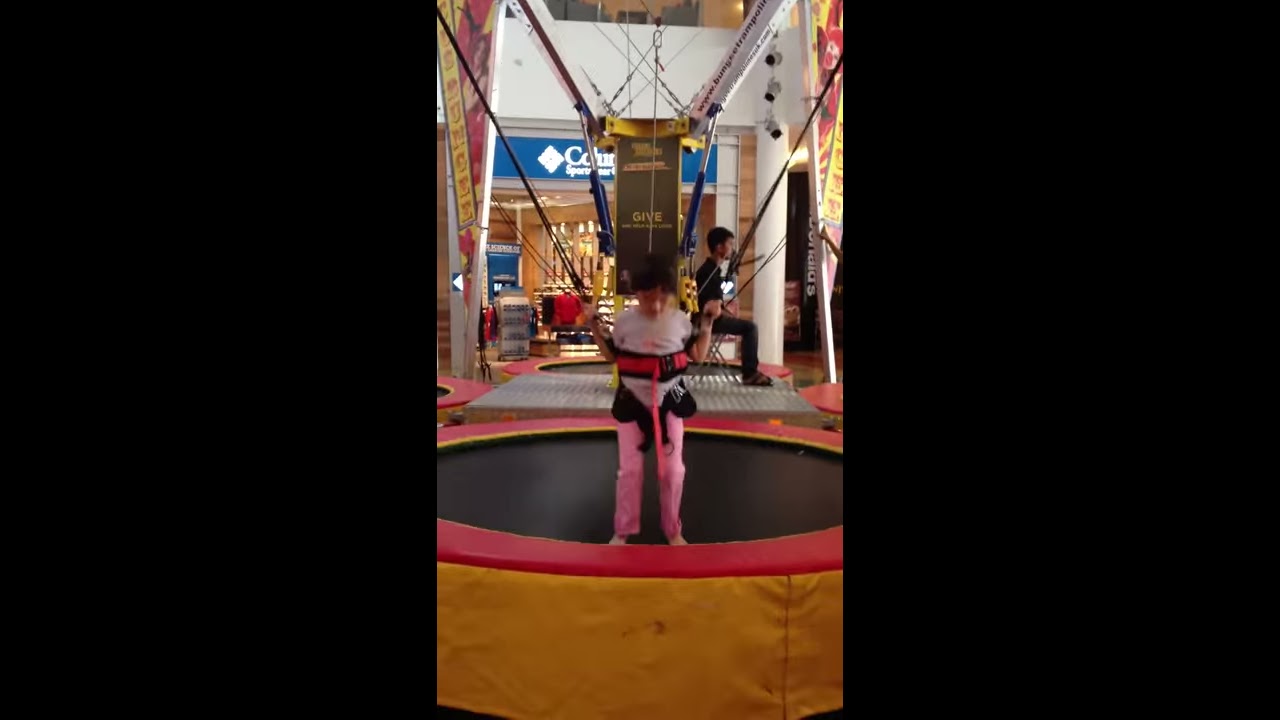This photograph, taken in portrait orientation inside a kids' play area of a mall, captures a young child mid-activity on a trampoline. The child, dressed in a grey (or white) shirt and pink pants, stands securely on the black central part of the trampoline, which features pink and yellow borders. The child is equipped with a black harness, secured by a red belt, and is holding onto several black ropes attached to the ceiling, ensuring safety. This setup appears to be part of a bungee jump or high-jump trampoline attraction. In the background, several elements of the mall are visible, including another trampoline area and a storefront with a partially visible "Columbia Sportswear" sign, suggesting the setting is within a commercial area. Vertical black strips frame the left and right sides of the image, likely part of the play area’s enclosure.